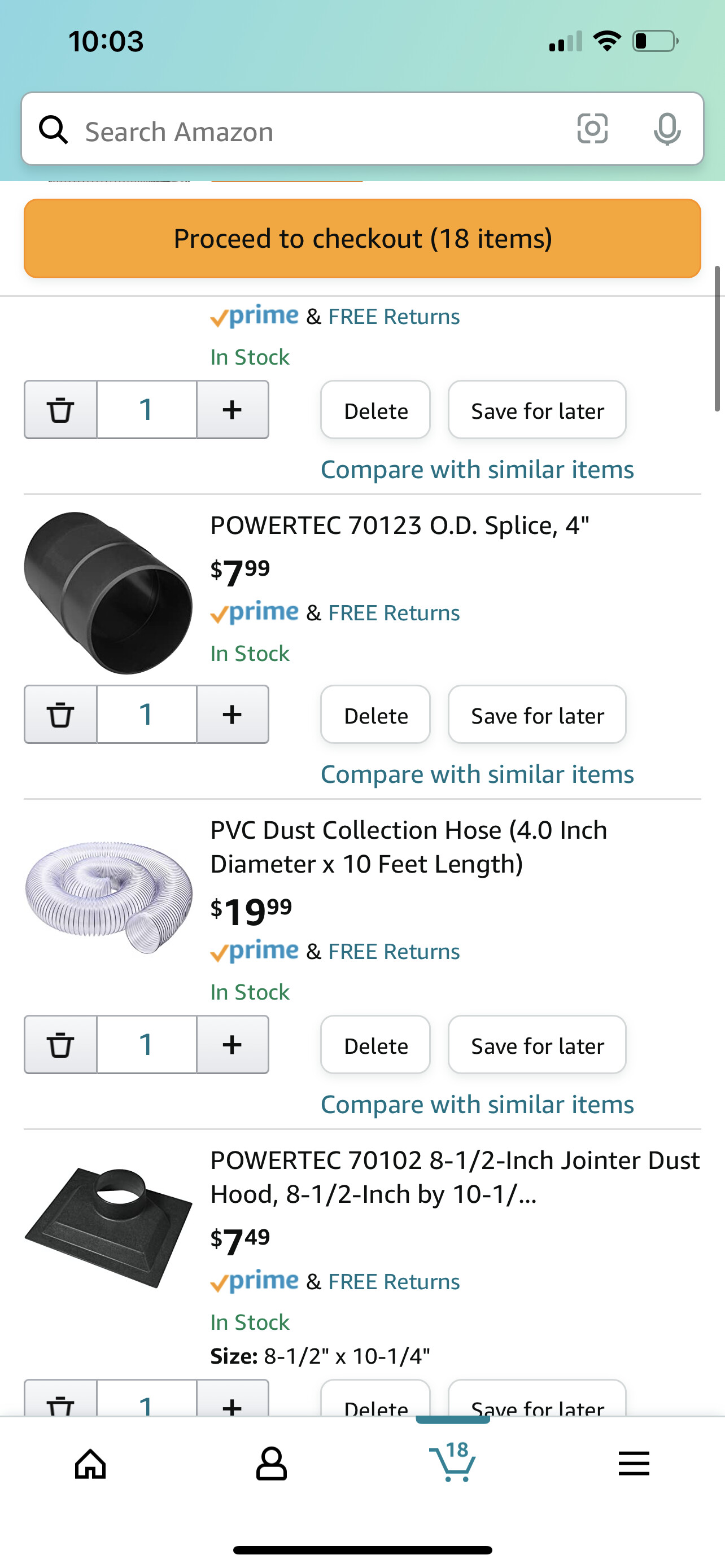Here’s a detailed and cleaned-up caption for the described image:

---

This screenshot displays the mobile version of the Amazon search page with a blue-green border at the top. The time, 10:03, is shown on the upper left-hand corner, whereas the upper right-hand corner indicates two bars of cell phone signal, a Wi-Fi icon, and a nearly empty battery. A long, horizontally-placed search bar, labeled "Search Amazon" in the center and featuring a camera icon and a microphone on the right, sits at the bottom of the blue section.

Below the search bar is a yellowish-orange rectangular button with rounded corners that reads "Proceed to Checkout. 18 items" in black text. Underneath this button, there are labels for "Prime" and "Free Returns."

The items listed in the cart include:
1. **Powertec 70123 OD Splice 4"** priced at $7.99, labeled with "Prime" and "Free Returns," and marked as in stock. The product image depicts a black, tubular object resembling a camera lens, facing diagonally to the left.
2. **PVC Dust Collection Hose, 4.0-inch diameter by 10-feet length** priced at $19.99, also labeled with "Prime" and "Free Returns" and in stock. The product image shows a white, coiled hose resembling a swirl.
3. **Powertec 70102 8.5-inch Joiner Dust Hood, 8.5-inch by 10-1/4 inch** priced at $7.49, with "Prime" and "Free Returns," and in stock. The product image shows a black, square object with a round hole at the top, presented diagonally to the left with white visible underneath the hole.

--- 

This caption comprehensively describes the elements seen in the screenshot, ensuring clarity and detail.